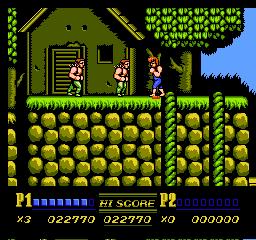This image depicts a vibrant, vintage video game screen, reminiscent of the 90s era, possibly resembling "Double Dragon." The scene unfolds on a grassy stone wall with a green house or structure in the background, suggesting where enemies might have spawned. It's a bright, colorful 8-bit aesthetic with a detailed blue sky and a large tree on the right, showcasing pixelated leaves. Three shirtless characters stand on the grass: the hero, resembling a Rambo-like boxer in blue pants, faces two identical enemies in green pants. At the bottom of the screen, game information is displayed: Player 1 shows an active score of 22,770 and health indicated by blue squares, while Player 2's info is visible but inactive, showing zero points. A high-score indicator is centrally positioned between the player stats, completing the retro gaming atmosphere.